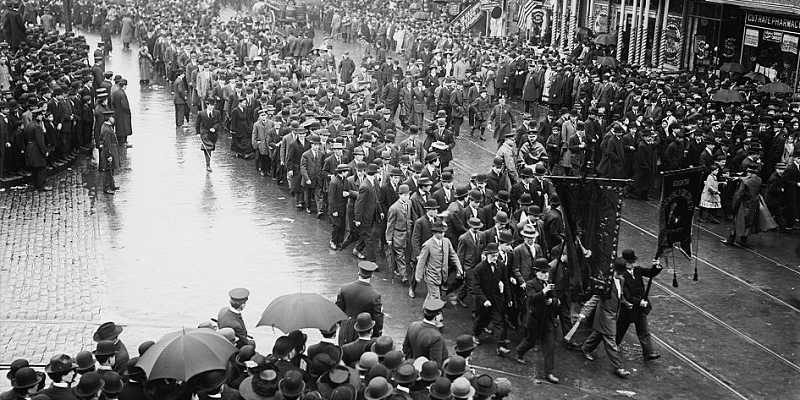In this evocative black and white photograph, we are transported back to a rainy day in a 1920s city, where a procession winds its way down the cobblestone streets. The scene is vibrant with the energy of a parade, despite the dreary weather. At the forefront, two men proudly carry banners, leading a group of men predominantly dressed in jackets, ties, and a variety of hats, mostly derbies and a few fedoras. The depth of the photograph reveals a wet street, its slick surface reflecting the steady rain.

In the foreground, police officers stand vigil, maintaining order in front of a crowd of onlookers. To the left side of the street, another group of men watches intently, while on the right side, people huddle under umbrellas on the sidewalk in front of buildings with storefronts—one notably marked "Pharmacy" in the top right corner. Central to the street are trolley tracks that bisect the scene, guiding the viewer's eye through the tableau of history and human activity. The intricate details of the image, from the attire of the participants to the urban elements of the setting, create a vivid snapshot of life during that era.